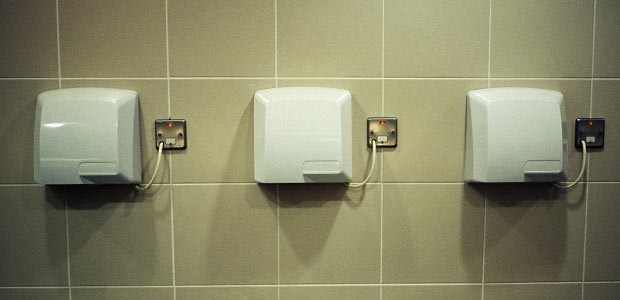The image depicts the wall of a public restroom lined with three equidistant white hand-drying machines mounted against large tan, tiled surfaces. Each machine is plugged into a square silver outlet, indicating them being powered on. These square-shaped devices feature a small, vent-like flap or handle on the lower right-hand corner, which is where you place your hands to activate a powerful stream of warm air designed to dry them quickly. The lack of text or instructions leaves their exact function somewhat speculative, but their design and context strongly suggest they are air dryers used after handwashing.